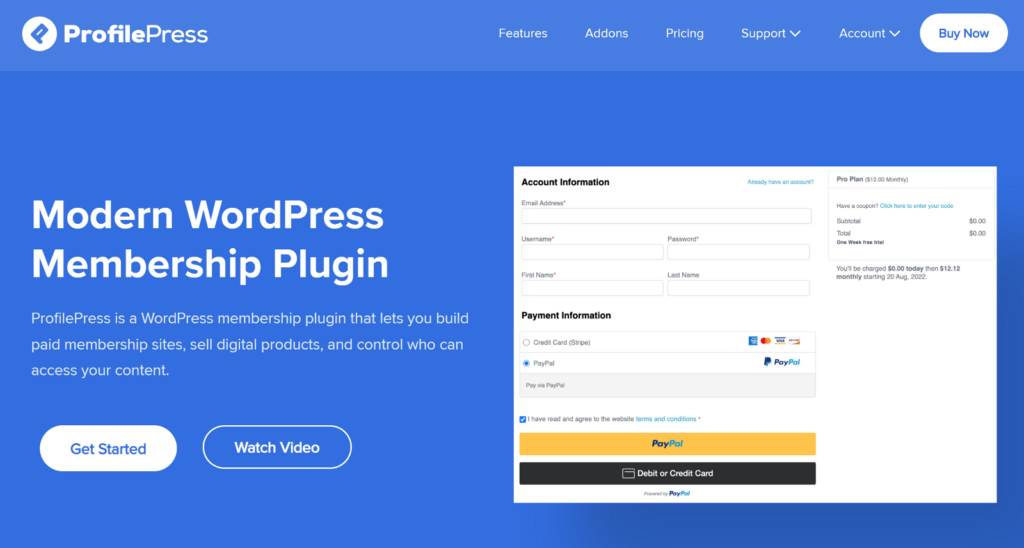The image is a rectangular banner oriented horizontally. At the top, there is a bluish border with white text that reads "Profile Press." To the left of "Profile Press," a small white circle features a flag icon. Midway across this border, the word "Features" appears, followed by "Add-ons," "Pricing," "Support" with a drop-down arrow, and "Account" also with a drop-down arrow. Further to the right, there is an oblong white button containing the text "Buy Now."

The next section of the image has a darker blue background, covering the remainder of the banner. On the left side of this section, large white text proclaims "Modern WordPress Membership Plugin." Below this, in smaller font, it adds, "Profile Press is a WordPress membership plugin that lets you build paid membership sites, sell digital products, and control who can access your content."

Continuing downward, there is a white button labeled "Get Started" and a blue button outlined in white with "Watch Video" written in the center. On the right side of the banner, a white box titled "Account Information" appears, prompting users to enter their email address, username, password, and first and last name.